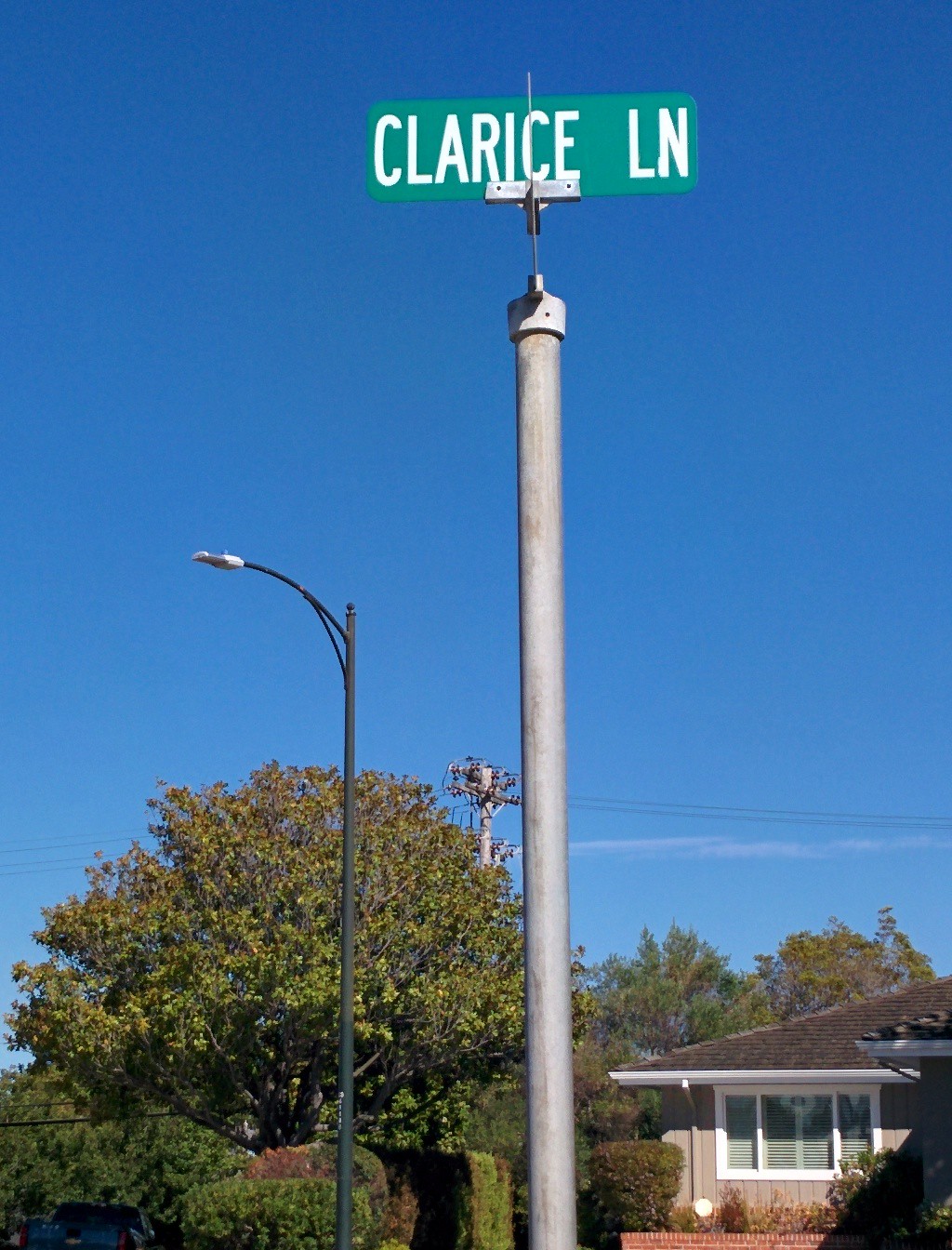In this contemporary modern photograph, the central focus is a street sign reading "Clarice Lane," mounted on a silver, gray-colored metal pole that spans almost from the top to the bottom of the image. To the left of the street sign stands a street light with a darker gray metal pole. The street sign and the street light are prominently featured against a vibrant blue sky that occupies the top three-quarters of the frame. 

In the bottom right-hand side of the photograph, a partial view of a house is visible. The house features a light gray facade, white-framed windows with three window panes each, and white gutters lining the roof. Though the front door is outside the frame, a window and some of the architectural details of the home are clearly captured. In front of the house, a brick planter hosts well-manicured shrubs and various plants, adding a touch of greenery to the scene.

The background of the photograph includes additional foliage, with a variety of shrubs and trees from the surrounding neighborhood adding depth and context to the serene suburban setting.